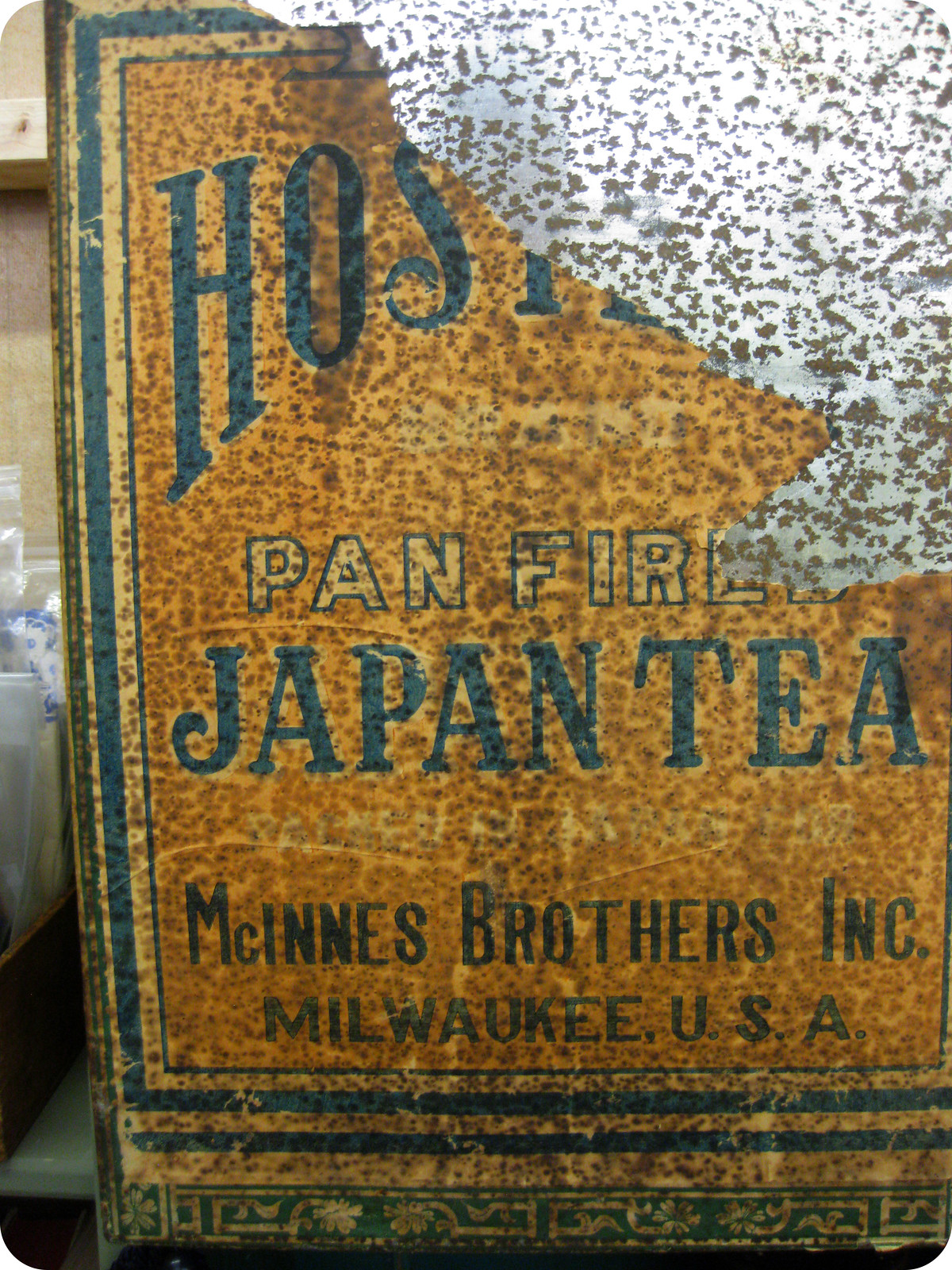This image depicts a close-up of an extremely old and faded sticker on what appears to be a tin can or box, potentially viewed through glass due to a visible reflection on the left side. The top right corner of the label is particularly worn and partially torn off, revealing white and gold speckles, with the gold speckles originating from the sticker itself. In green text, the label reads "H.O.S." and seems to say "hostage," although it's cut off after the T. Below this, the remnants of the text "PAN FIRED" can be seen, with the "E" and "D" missing. Further down, in complete green text, it states "JAPAN T." The label continues with "McInnes Brothers Incorporated," followed by "Milwaukee, USA," both in black text and fully visible. The green-bordered sticker is heavily stained and decorated with ornate embroidery along the edges, attempting to lend a fancy appearance despite its substantial wear and discoloration. The can itself features a yellow background with blue and tan borders, showcasing a mix of blue, light yellow, and black text amidst its vintage charm.